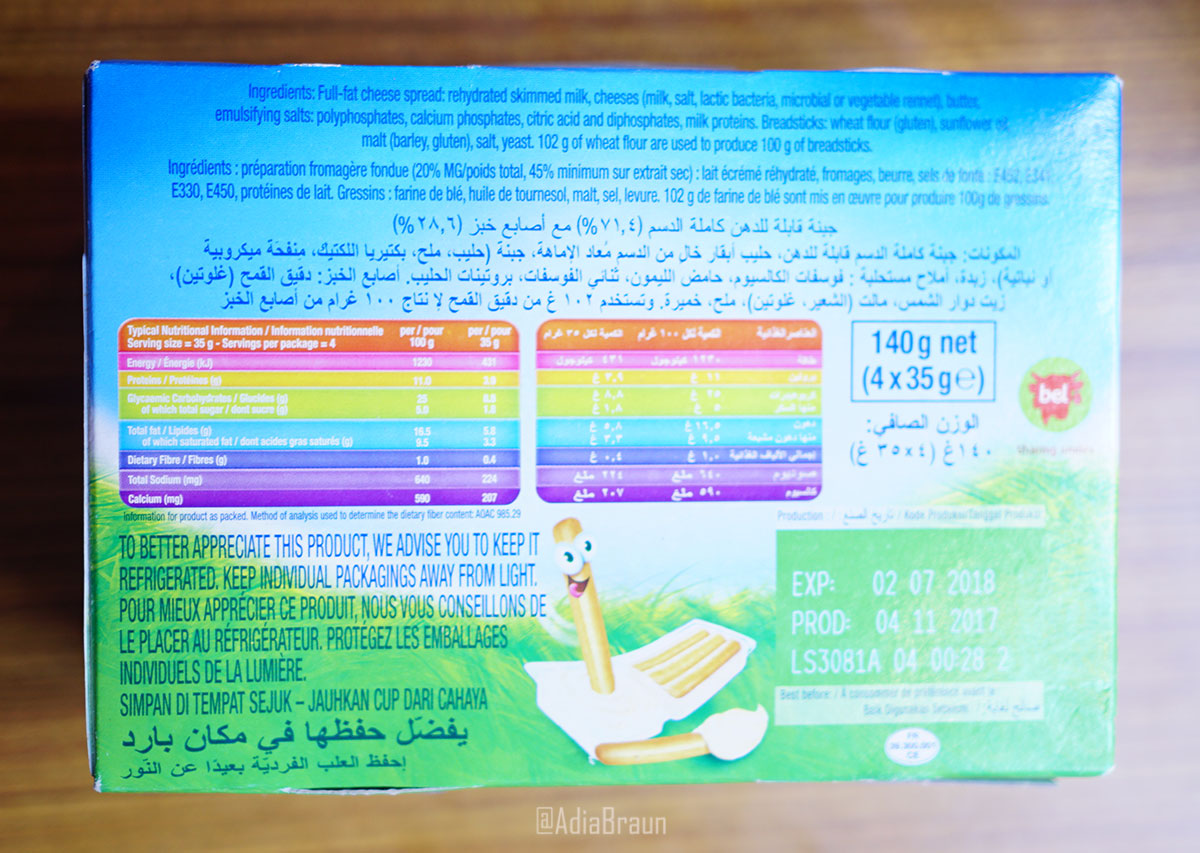The photograph showcases the back of a package set against a light brown wooden background with prominent dark brown veins. The label on the package is a large rectangle with a gradient background, transitioning from blue at the top to white in the center, and finally to green at the bottom quarter. 

At the upper section of the label, there are several rows of text in blue writing. Below this section, Chinese characters span several rows. Further down on the left side, there is a vertically aligned rectangle containing rows of white text, each row highlighted with different colors: orange, pink, yellow, light green, blue, and purple. Adjacent to this, on the right, is a smaller rectangle with a similar colorful format.

To the right of these rectangles, a blue-outlined box reads "140GNET". Below this, it says "4X35GE" enclosed in parentheses. Underneath the colorful rectangles on the left side, more blue writing can be found. To the right of this writing is a peculiar depiction that resembles a yellow-orange hot dog standing upright within a white square, accompanied by a white-tipped scoop with a yellow-brown handle, likely representing an ice cream scoop. Additional writing is present in the lower right-hand corner of the label.